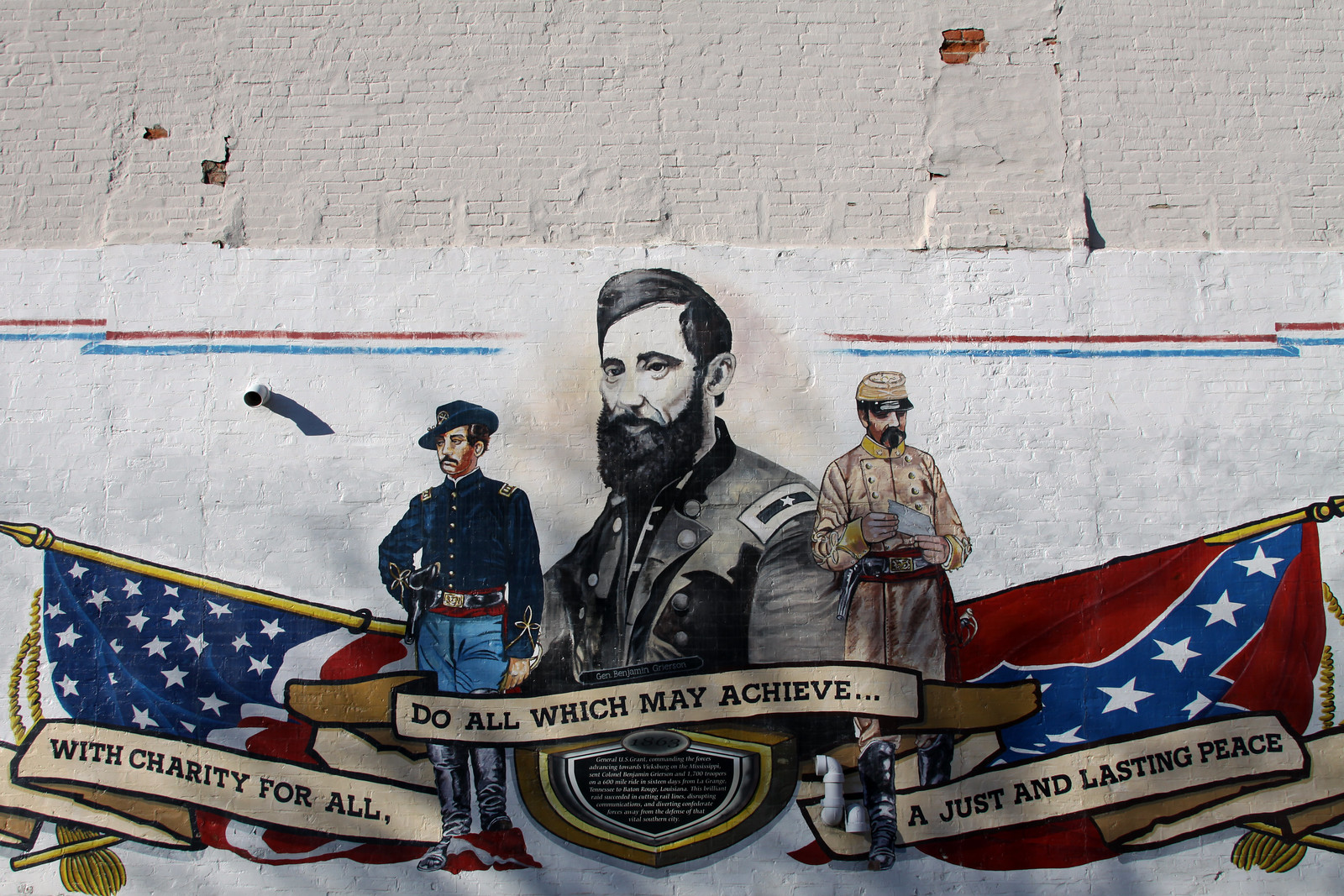This image depicts a detailed mural painted on a beige and white brick wall, with the paint chipping off at the top half, revealing a brick design underneath. The focal point of the mural features three historical figures: the central figure in a black and white image with a prominent beard, possibly a president, surrounded by two soldiers in historical uniforms. The soldier on the left is dressed in a Union blue suit and features an American flag, while the soldier on the right is clad in a Confederate light brown suit with a Confederate flag beside him. Below these figures, various banners convey a unified message of reconciliation and peace. The left banner reads "with charity for all," the central banner states "do all which may achieve...," and the right banner concludes with "a just and lasting peace." Additionally, there's an unreadable text on a small plaque at the center bottom of the mural.